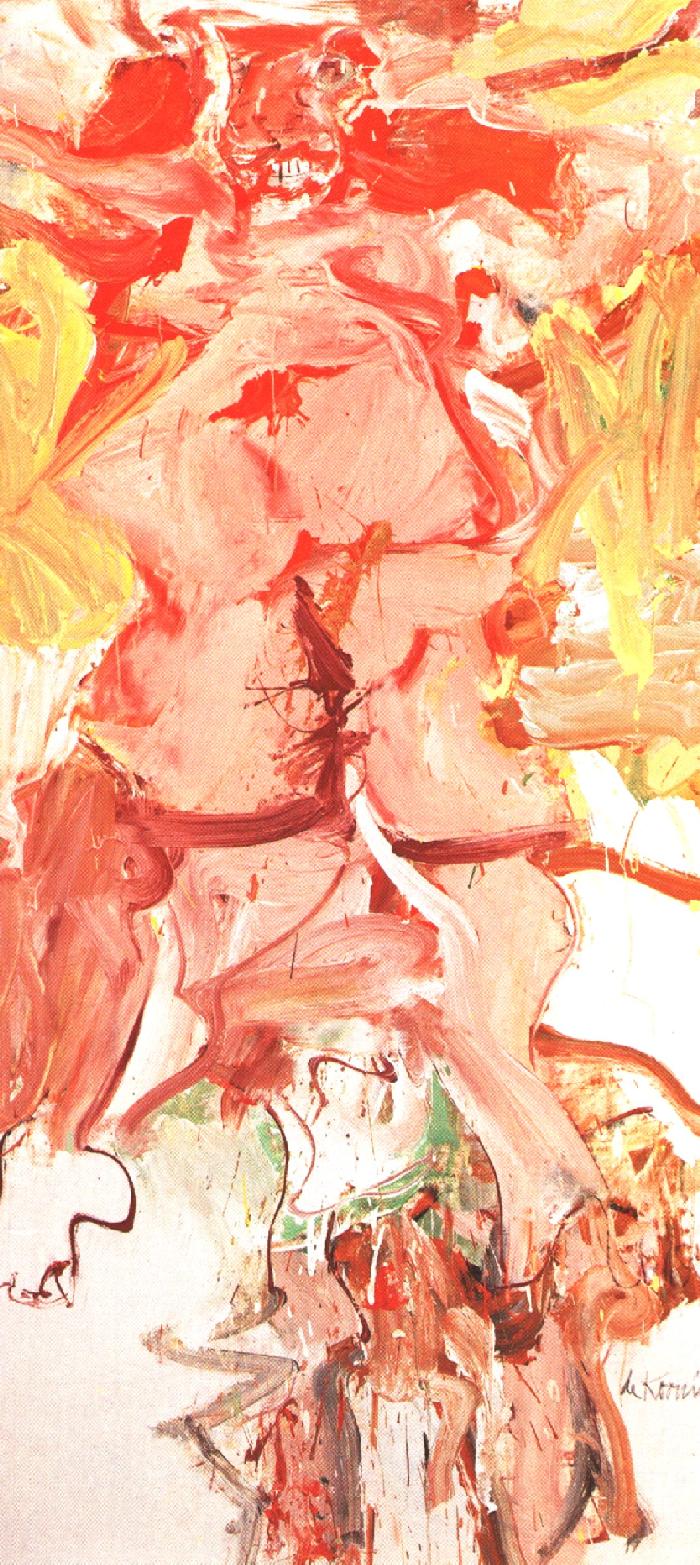In this abstract painting, which is oriented in portrait mode, vibrant colors dominate the canvas, creating an intricate and perplexing composition. The central focus of the artwork is a large, red smear that extends vertically from the top to the bottom, flanked by yellow splotches. Throughout the painting, various shades of orange, dark reddish-pink, light pink, and white intermingle, with subtle hints of green and brown near the bottom of the piece. The background prominently features white, adding contrast to the vivid colors. Amidst this colorful chaos, some viewers might discern a vague human or beast-like figure with an obscure face towards the top center, a flesh-colored body, and two indistinct legs. There may even be a suggestion of femininity, potentially identifiable by shapes resembling breasts. The brush strokes vary in direction, with some appearing vertical, others horizontal, and some even swirled. In the bottom right-hand corner, a nearly indecipherable signature, possibly reading "L-E-K-O-R-N-I," finalizes the composition, adding a personal yet enigmatic touch to the artwork.